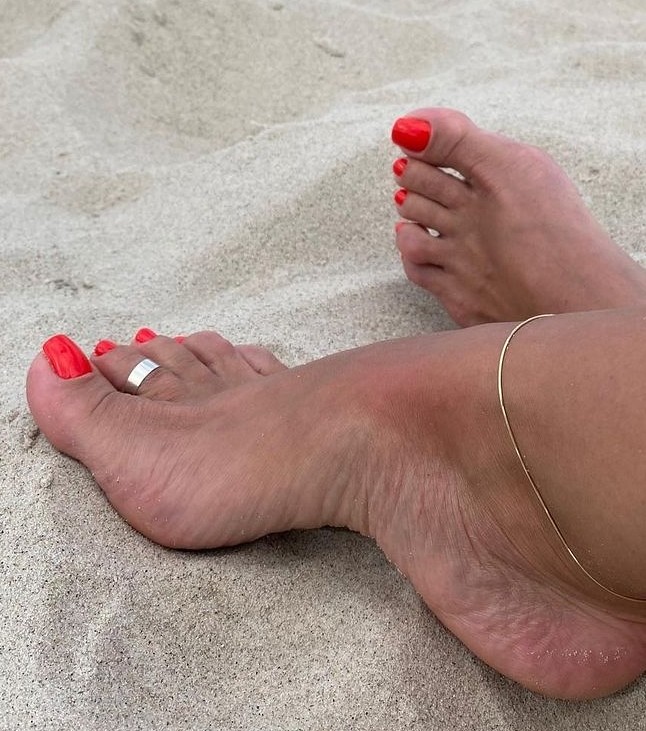This is a detailed photograph taken during daytime at a beach, showcasing a pair of crossed feet on light-colored, speckled sand. The right foot, with coral-orange painted toenails, is crossed over the left foot, which also has similarly painted toenails. The right ankle is adorned with a delicate gold or silver anklet, and the second toe on the right foot features a silver toe ring. The sand beneath and around the feet appears clean and has natural ridges, with shadows cast by the slightly elevated right heel, indicating the foot is pressed into the sand. The scene is bathed in daylight, highlighting the colors and textures of the feet, jewelry, and sand.